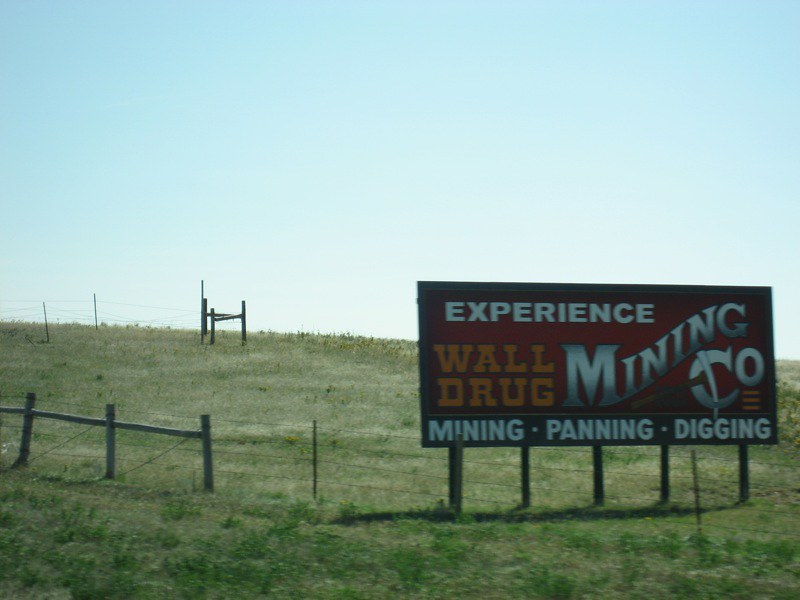This image captures a billboard set in a serene, open field, supported by rustic wooden poles. The field is lush with green grass, typical of a countryside locale, and seems to be positioned near a road, as evidenced by the wire fence that runs horizontally across the foreground of the scene. The billboard is located on the inner side of the fence, suggesting it might be on private property, potentially owned by a local farmer or leased from one.

The rectangular billboard features an eye-catching red background framed by a black outline. The text is styled in an old-fashioned, saloon-style font, adding a nostalgic charm. The top of the sign prominently displays the word "Experience" in bold white letters. Below it, the phrase "Wall Drug" stands out in vibrant yellow. To the right, the words "Mining Co." appear in a silver hue, crafted to give a metallic effect, accompanied by an illustration of a pickaxe, symbolizing the mining theme.

At the bottom of the sign, white text on a black background spells out "Mining, Panning, and Digging," suggesting an interactive adventure. This billboard likely advertises a unique roadside attraction where visitors can experience the thrill of historical gold mining activities. Such attractions allow guests to immerse themselves in the practices of the old gold rush era—panning in streams, digging, and perhaps mining for treasures—offering both entertainment and a window into the past.